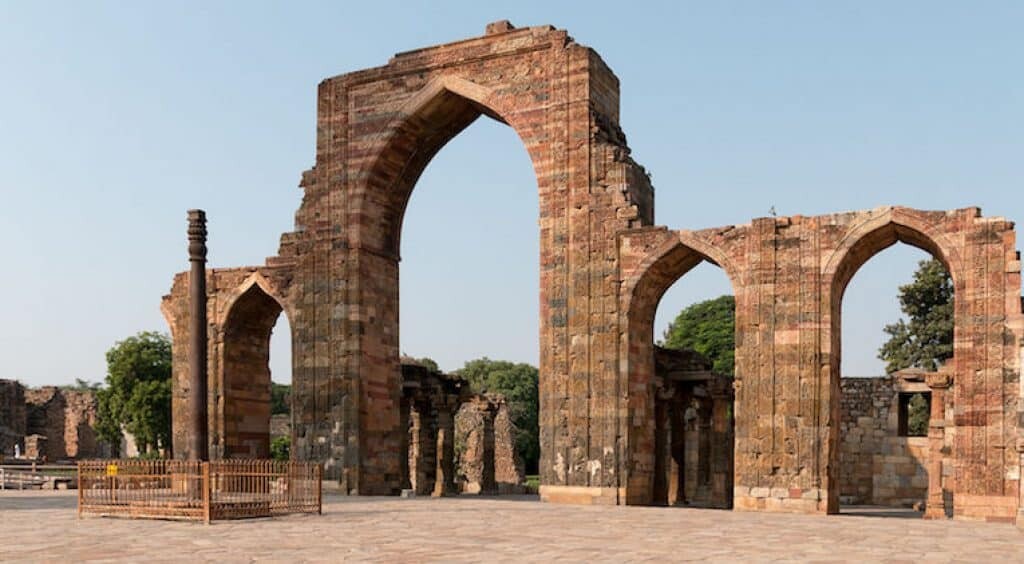This outdoor photograph captures what appears to be the remnants of an ancient, slightly rundown structure with a striking resemblance to a Greek Coliseum's architectural style. The centerpiece of the image is a series of four rounded archways made of darker reddish-brown bricks, which exhibit wear and age, suggesting abandonment for decades if not centuries. The largest archway stands prominently in the center, with its top coming to a soft curve. Through these archways, a light blue, cloudless sky is visible, adding a serene backdrop to the scene.

In front of the archways lies a pole or lamppost, encased in a small, rust-colored metal fence, approximately two and a half feet high, possibly meant to protect the structure from visitors. The ground beneath is composed of a reddish-pale-white tiled stonework. The image's left side reveals a glimpse of a street, indicating urban proximity.

Behind the arches, several trees lend a hint of nature and further frame the ruins, adding depth to the image. The background features more faded, dilapidated architectural elements, reinforcing the historical context of the place. The clear, bright sky enhances the overall clarity and sharpness of this picturesque yet melancholic scene.